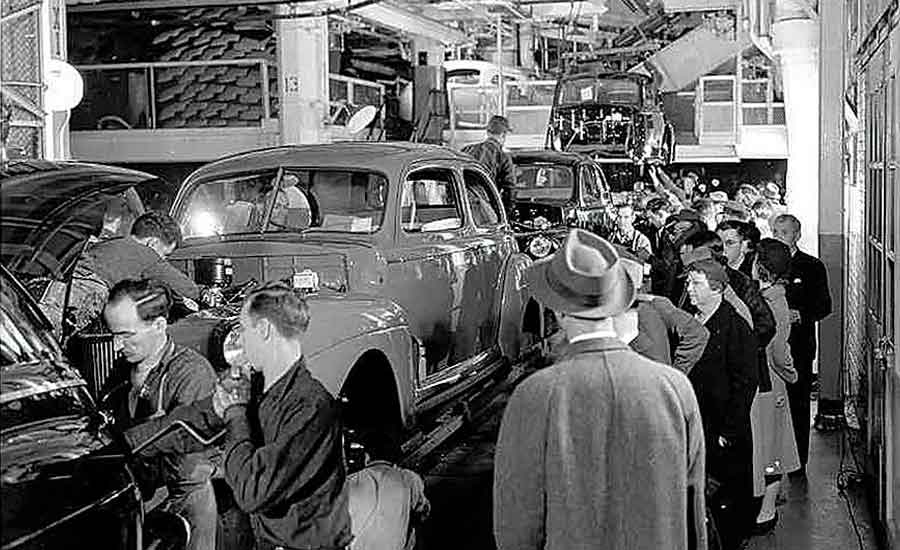This black and white photo, likely from the mid-20th century, captures a bustling scene inside an industrial automobile factory. Centered on an assembly line, the image shows several men working on cars in various stages of assembly, from partially built frames to nearly complete vehicles, elevated at about waist height. In the foreground, a man with his back to the camera and wearing an old-fashioned hat oversees the activity. To the left, two workers are focused on the back of one of the vehicles. On the right, a crowd of onlookers, including one woman in a light gray coat among mostly dark-coated observers, watch the assembly process intently. The background is filled with additional cars and industrial structures, giving the entire scene a sense of organized chaos indicative of a busy manufacturing environment. This detailed moment, possibly documenting a significant event such as the opening day of the plant with reporters present, highlights the era's industrial prowess and the communal interest in automotive innovation.